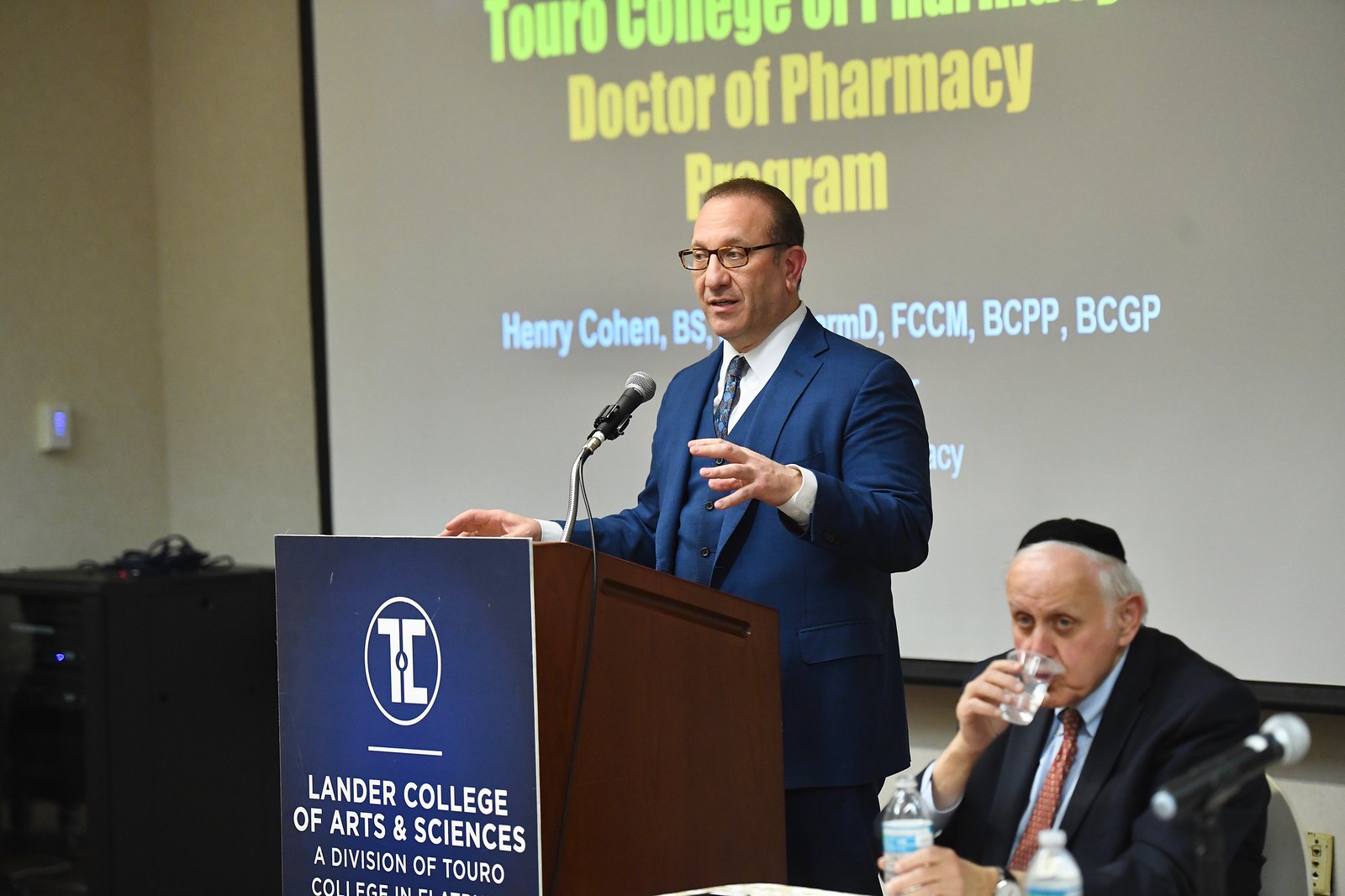The image depicts an indoor event at Lander College of Arts and Sciences, a division of Touro, featuring a man standing behind a dark brown wood podium with a blue sign on the front that reads "Lander College of Arts and Sciences, a division of Touro." The speaker is wearing a blue suit, a white collared shirt, and a blue tie, while addressing an audience through a microphone attached to the podium. He is holding one hand up and wears glasses. 

Behind him, a projection screen displays a partially visible slide, with readable text including "Doctor of Pharmacy Program" in yellow, "Henry Cohen BS," and additional credentials "FCCM, BCPP, BCGP" listed in white text. The image also includes another man, presumably older, seated at a table next to the podium. This man is dressed in a dark suit with a blue collared shirt and a red tie, and he is wearing a yarmulke. He appears to be holding a bottle of water in one hand and drinking from a glass with the other. The walls of the room are painted white, providing a neutral backdrop for the formal event.